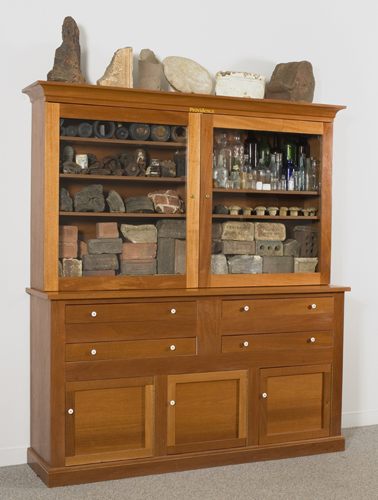This photograph captures an antique wooden hutch situated in a white room with short gray carpeting. The hutch is composed of two distinct parts. The lower section features a combination of cabinets and drawers: three doors at the bottom center, flanked by two drawers on either side. While the contents of the closed cabinets remain hidden, they might typically store items like silverware, pots, pans, or serving dishes. 

The upper section of the hutch showcases two large glass-fronted cabinets. The left cabinet contains four shelves, while the right has three. The shelves hold an eclectic collection of various-sized rocks, bricks, concrete blocks, cinder blocks, and glass bottles, possibly including historical artifacts such as old building materials or labeled collectibles. Atop the hutch, there are six substantial rock formations or small boulders, adding a unique and rugged aesthetic to the piece of furniture.